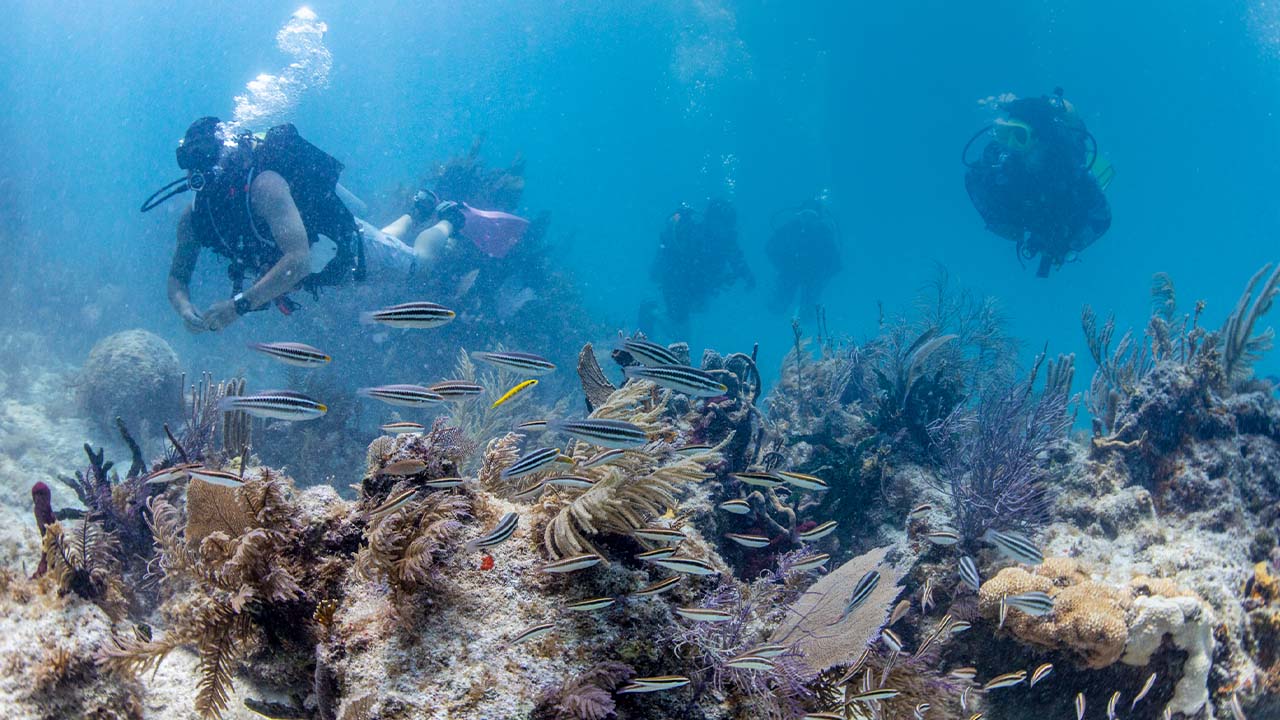A crystal-clear underwater photograph captures a vibrant coral reef teeming with marine life and four scuba divers exploring the ocean depths. Two scuba divers are in the foreground, one on the left wearing pink fins and seemingly male, while the other is to the right. Both are positioned closer to the camera, with the remaining two divers hovering in the background. The scene is bathed in natural light, illuminating the coral formations and a variety of sea plants, including kelp and polyps. A school of black and white striped fish, approximately 6 to 10 inches long, along with occasional yellow fish, swim leisurely nearby. Numerous air bubbles trail upward from each diver's mask, enhancing the sense of movement and vitality in this serene underwater snapshot. The palette consists of muted tans, blacks, and whites, highlighting the natural beauty of the seabed.